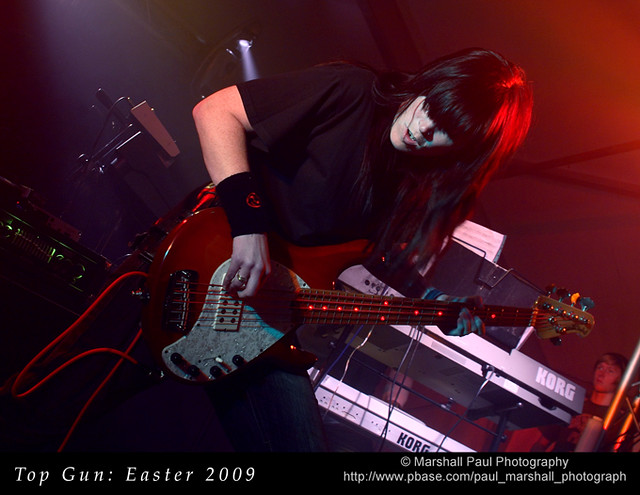The image captures a dynamic moment on stage during a music concert, featuring a male musician with long, dark hair highlighted in red by stage lighting. He is playing a red electric bass guitar with a white marbled pick guard, from which a red cord extends. Clad entirely in black, including a black sweatband with a red symbol around his wrist, he stands in front of two tiered Korg keyboards. The stage background is dark, enhancing the dramatic red lighting that accentuates his hair. To the right, partially visible, is the arm of the keyboard player, who also wears dark clothing. At the bottom of the image, a banner reads "Top Gun Easter 2009" in white text, with credit for the photograph given to Marshall Paul Photography, accompanied by a website URL. The overall atmosphere is intense and focused solely on the performing artist.